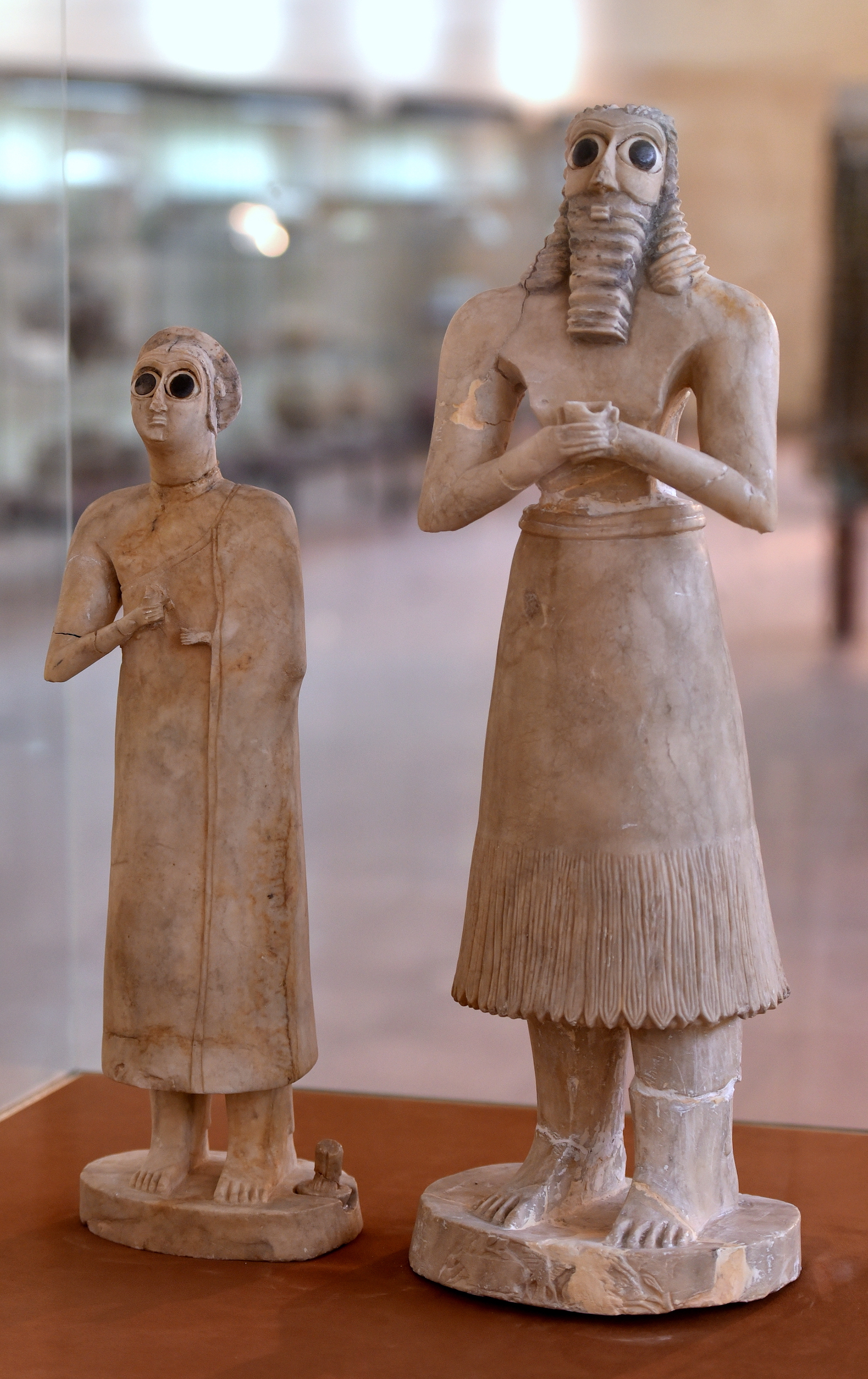This is a vertically rectangular full-color photograph taken indoors, likely in a museum setting. The background is indistinct, with blurred shapes in the distance and potential natural light filtering through windows on the top left. The display features two carved stone figures with distinct stylistic elements suggesting an ancient civilization, possibly Assyrian. The figures, appearing brown in color, are positioned on a brown wooden pedestal, encased in glass as indicated by a crease visible on the left side.

The left figure is notably smaller, adorned in a long robe that covers its body down to its bare feet, and has one visible arm. Both figures share a striking feature: massive black eyes with large pupils dominating their eye space. The right, taller figure has a long square-cut beard, and curly hair that cascades back behind its head onto the shoulders. Unlike the smaller figure, this one wears a waist skirt extending to mid-calf, leaving his chest exposed. Each detailed element enhances the mysterious and ancient aura of this museum display.